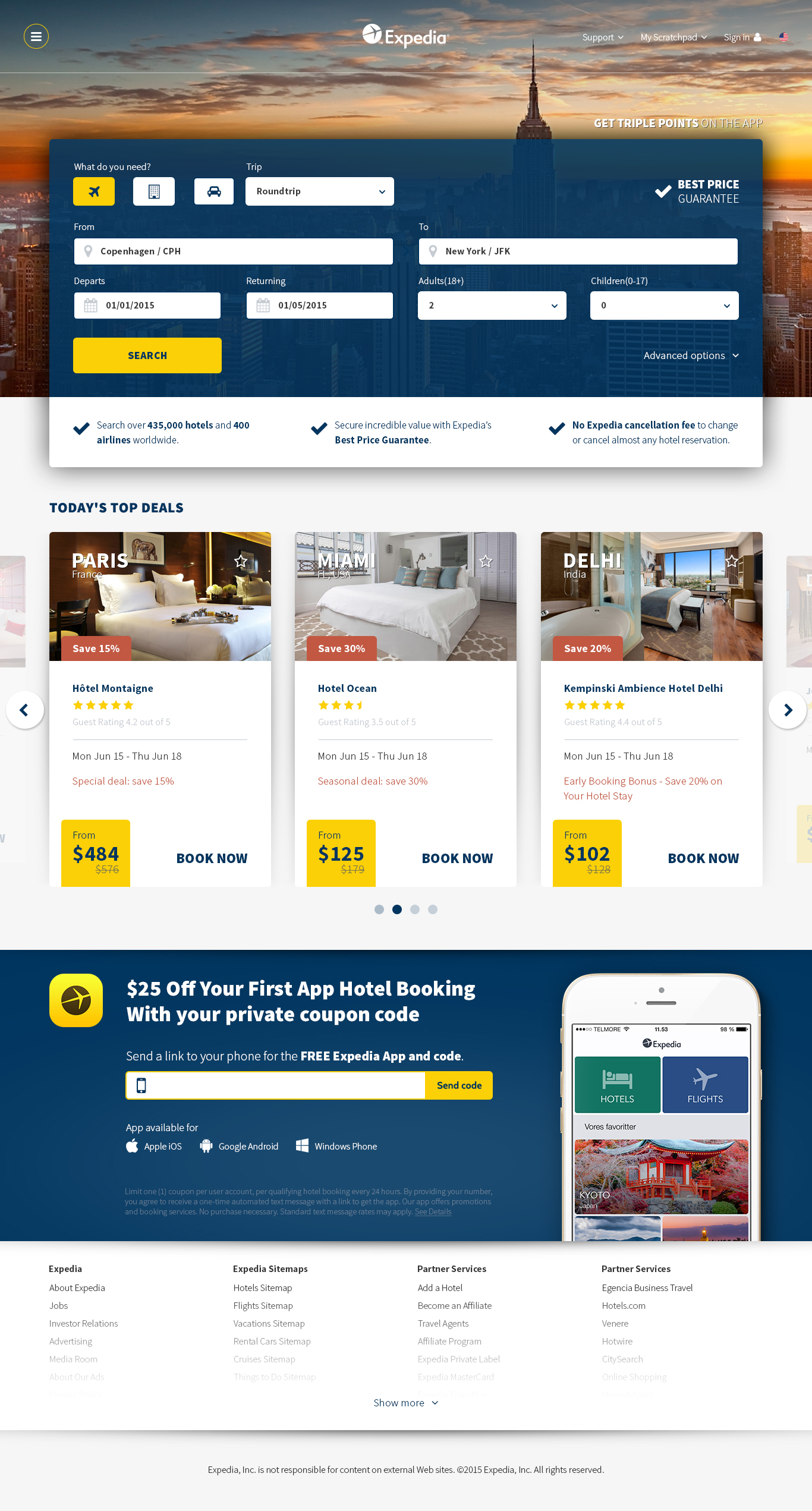This image from Expedia displays a visually appealing and user-friendly interface designed for travelers. The background showcases a picturesque scene, featuring a steeple at the center, bathed in a beautiful sunset, flanked by images of buildings on both sides. The top section of the website is dedicated to a search bar where users can input their travel details. 

Once the necessary information is entered, the 'Search' button activates the site's powerful search functionality. The interface includes helpful icons with check marks guiding users through the process. Highlighted prominently are "Today's Top Deals," showcasing impressive offers. 

The first deal features Paris, priced at $484, with a five-star rating, and a prominent 'Book Now' button. The next deal is for Miami, available for $125 with a four and a half star rating, also with a 'Book Now' option. A third offer for Delhi is listed at $102, boasting a similar star rating and booking option. 

Additional perks include a promotion offering $25 off the first app hotel booking with a private coupon code. This offer is illustrated with an image of a phone, emphasizing the convenience of booking via mobile. The white background and strategic use of colors, such as blue for the 'Book Now' buttons, alongside clear, black informational text, ensure all information is easily accessible and visually engaging.